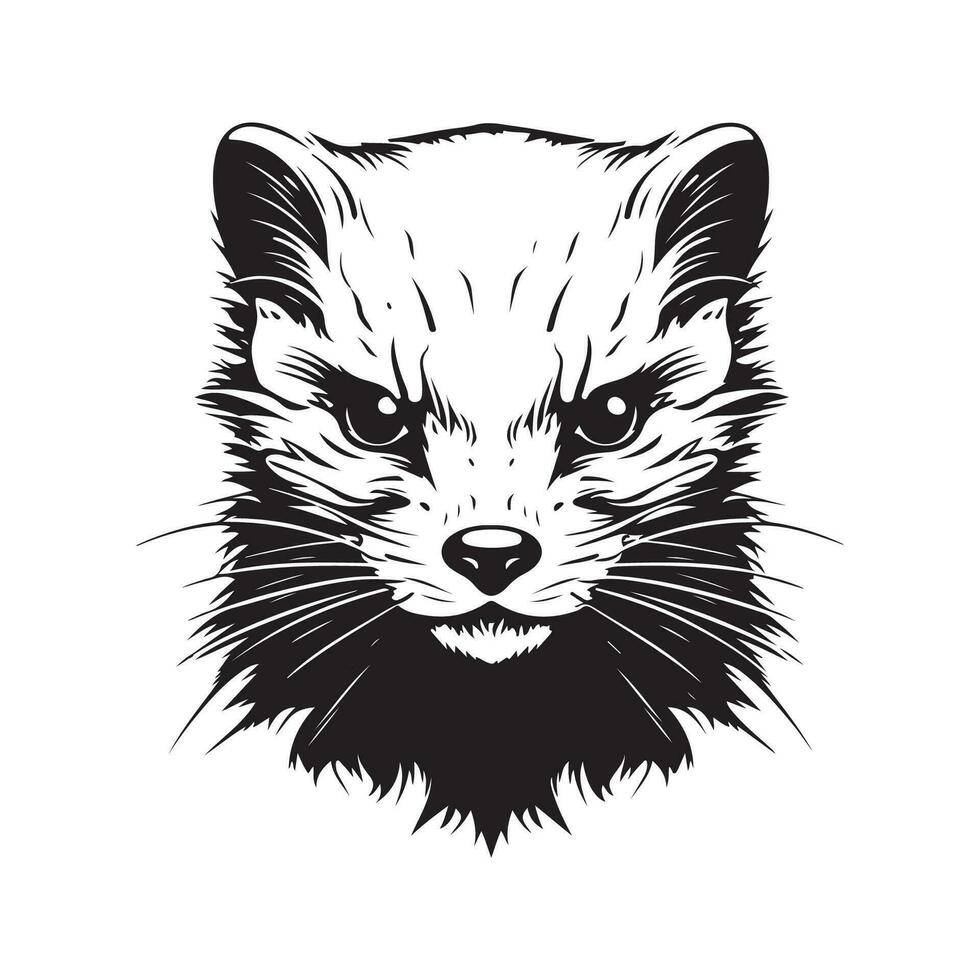The image is a detailed black and white digital illustration of a small mammal, likely resembling a stoat or a similar animal like a ferret or weasel. The creature's head faces directly toward the camera, captured from a central perspective that accentuates its fierce and intense gaze. Its face forms an upside-down triangle, with the ears positioned at the top corners. These ears are small, circular, and lack pointed tips. The mammal's striking eyes are depicted as black marbles with reflective highlights in their top right corners, adding a lifelike quality. The nose is button-like, also black with a reflective surface, accentuating its glossy texture. Numerous white whiskers with black outlines spring from the nose, further defining its expressive character. The illustration employs black wispy lines around the head to represent fur, merging with the white background to enhance the furry look. Overall, the image effectively uses black lines and fields of color to create a textured, lifelike portrayal of this small mammal within a stark white background.